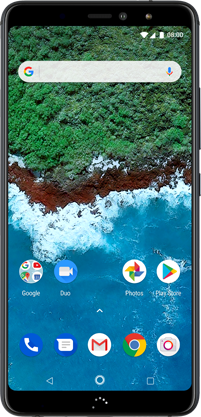A detailed screen capture of an iPhone showcases a black-cased device with the familiar top ribbon icons for battery life, signal strength, and connectivity status. The iPhone's home screen displays an intricate aerial view of a shoreline as its background wallpaper. Centrally focused, the ocean occupies the lower half of the image, merging into the brown sandy coastline with visible breakers. The upper section of the shoreline is adorned with dense, deep green foliage.

The bottom half of the screen is neatly organized with app icons. The top row features four apps: Google and Duo on the left, followed by Photos and Play Store on the right. The bottom row contains five apps: the phone dialer icon, text messages, a central 'M' icon likely for a specific app, Google's search bar, and the camera icon on the far right. This screen capture effectively captures the visual aesthetics and organizational layout of an iPhone's home screen, complemented by a captivating coastal screensaver.